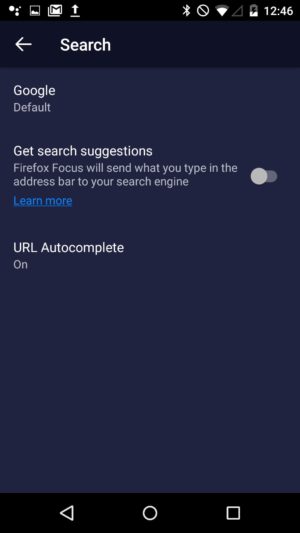The image features a user interface screen with a dark blue background. At the top, a black box contains a white square with an "M" and an upward arrow with a line beneath it, followed by the number "1246." 

Below this, another dark blue section includes a white left arrow symbol and a search bar with the text "Google default" indicating the default search engine. The text "Get search suggestions" appears, with an explanation that "Firefox Focus will send what you type in the address bar to your search engine." A white toggle switch indicates this feature is enabled. Additionally, there is an underlined "Learn more" in blue text.

Further down, the phrase "URL autocomplete on" is displayed, indicating that the autocomplete feature for URLs is active.

At the very bottom, another black box displays three icons: a left arrow, a circle, and a square, likely representing navigation and functionality buttons.

Overall, the screen details the search and autocomplete settings for Firefox Focus in a well-structured layout.